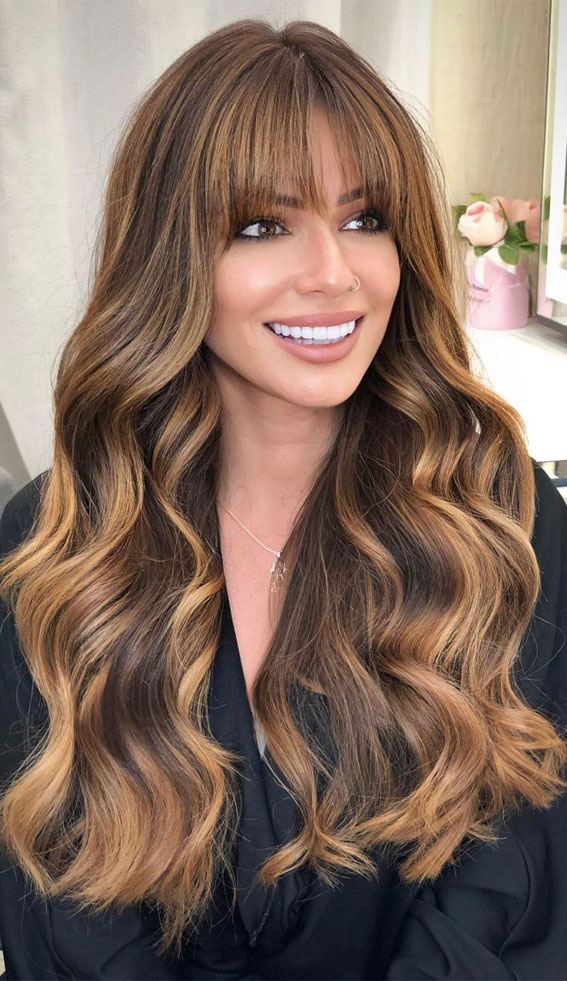The image features a woman with strikingly long, wavy brown hair adorned with light blonde highlights that cascade down to her chest or just below. Her hair is glossy and frames her face, which is characterized by brown eyes, a thin nose, and an unmissable, vibrant white smile, giving her an almost supermodel-like appearance. She exudes confidence and self-esteem, indicated by her bold, slightly plasticky smile. She is dressed in a black robe or smock over a v-neck shirt, accessorized with a silver necklace. She has a smooth complexion and long bangs, and she gazes off to the right, not directly into the camera. The image's background includes a white curtain, a tan wall, a flower in a pink dish, a white shelf, and possibly a mirror or window, although the back is somewhat washed out. The overall setting is bright, with the woman being the clear focal point of the photograph.